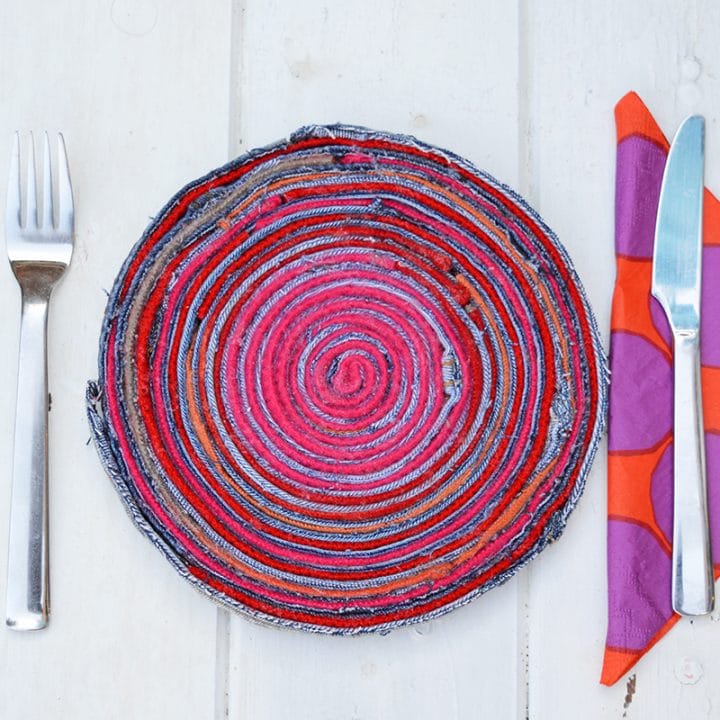This photograph captures a vibrant and eclectic place setting atop a white painted wooden slat background. At the center, a colorful, round woven placemat, resembling an intricate piece of pottery, is adorned with concentric spirals of pink, various shades of blue, red, and hints of orange. To the left of this striking centerpiece is a shiny silver fork, its four tines and thick handle elegantly flanged at the bottom. To the right, an intricately folded light orange napkin with dark orange-outlined purple circles lies partially out of the frame. Atop the napkin rests a slender silver knife, distinguished by a slightly curved indent on the left side of the blade. The overall composition blends a lively palette and a mix of textures, creating a visually arresting dinner setting.